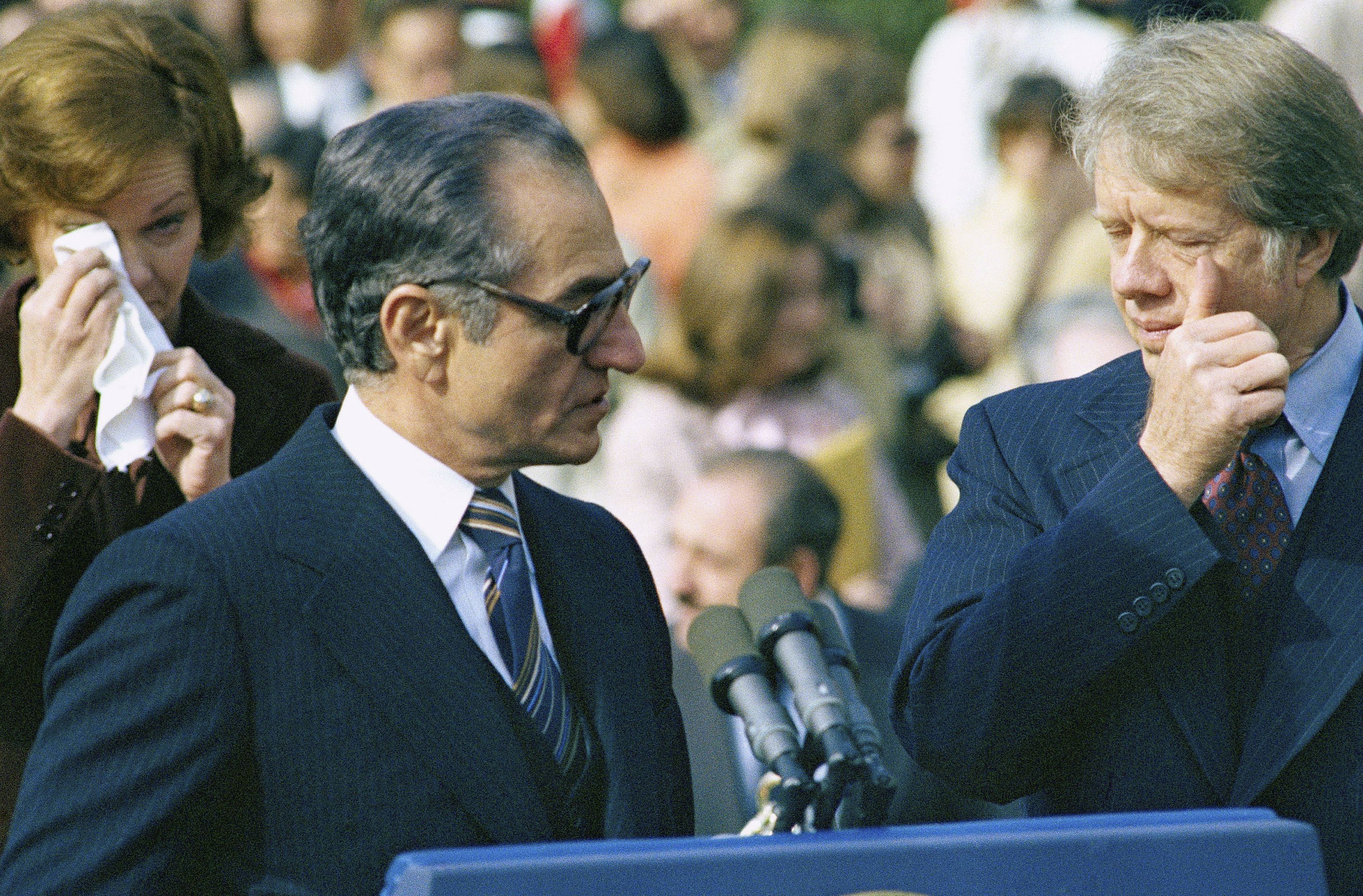This poignant photograph captures a somber moment, likely from the late 1980s, during a political speech involving former President Jimmy Carter and his wife, Rosalind Carter. At the forefront stands a man with thick-rimmed tortoiseshell glasses and graying combed-back hair, dressed in a blue striped suit with a striped blue tie over a white shirt. He is positioned at a podium adorned with four or five microphones, addressing the audience with a solemn expression. To his left, President Carter, also in a blue striped suit but distinguished by a purple foulard tie, is seen wiping his eyes in evident grief. Behind the speaker, Rosalind Carter, clutching a handkerchief, wipes tears away, further emphasizing the deep sorrow shared by the attendees. The blurred background reveals a gathering of people, contributing to the overall mournful and formal tone of the scene. The primary hues of blue, white, brown, and gray dominate the image, which exudes an air of collective mourning, suggesting the occurrence of a significant and tragic event.